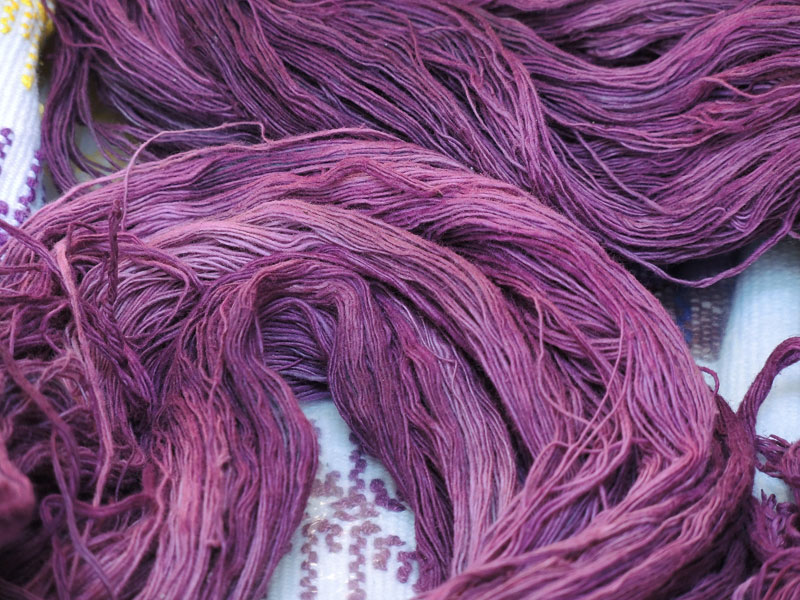This close-up image presents a detailed view of thick strands of yarn exhibiting varying shades of purple, although one description interprets it as red and possibly thin rope. The yarn is arranged in two distinct areas: one cluster at the bottom extending upward and then looping back down, and another large clump on top of the first, creating a sense of layered depth. The yarn appears to be fairly thick, almost resembling hair, and might be part of a larger item such as a wig or a scarf, though no clear connections indicate an assembled piece. The background features a white blanket with subtle yellow and purple colors, with some brown squiggly lines underneath that look like sewing machine stitching, adding to the intricacy of the scene.